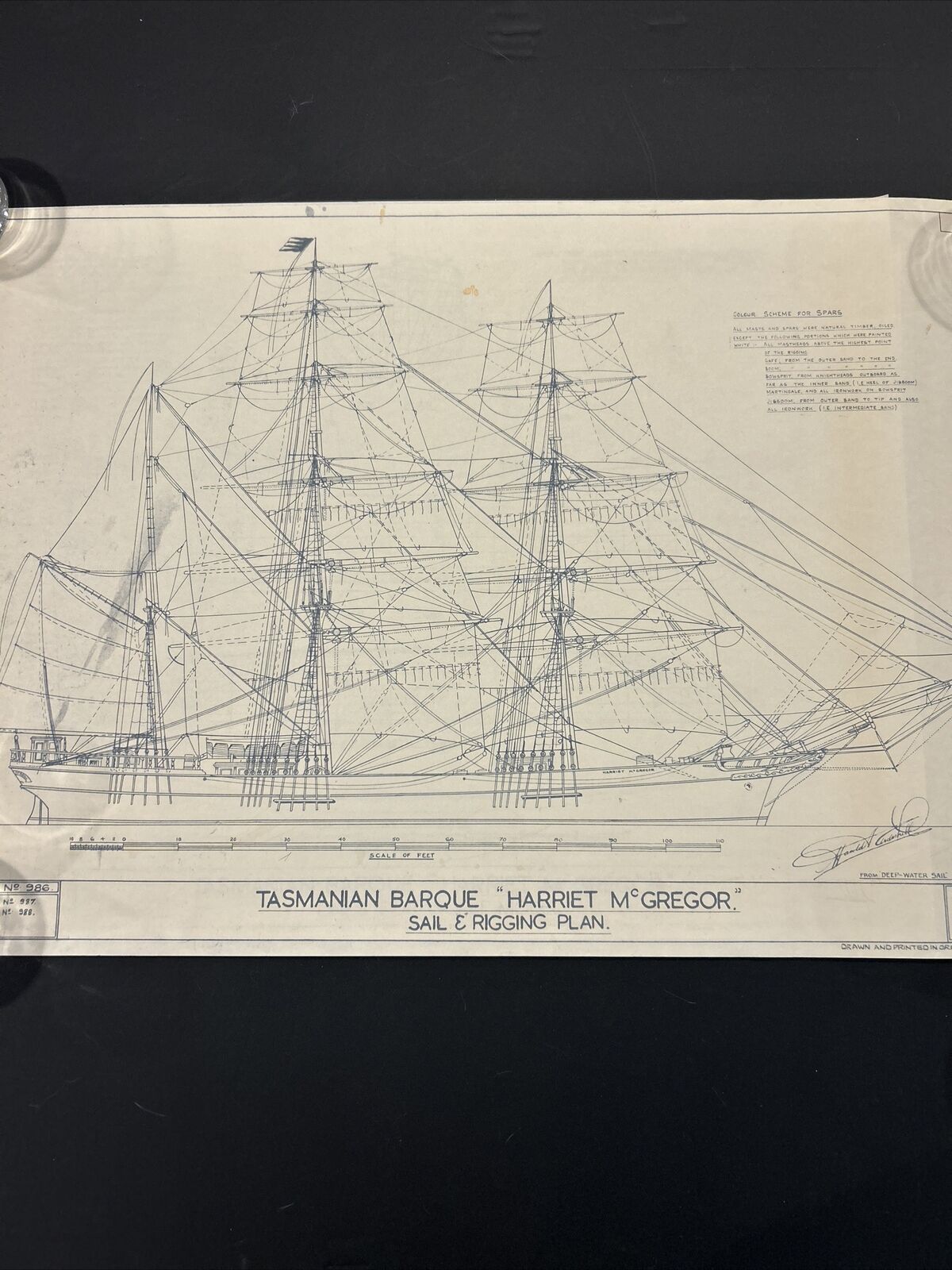This image is an intricately detailed, old-style architectural drawing of a large sailing boat, known as the Tasmanian Bark, designed by Harriet M. Greger. The blueprint, titled "Sail and Rigging Plan," features fine bluish lines on a plain white background and incorporates a range of scales likely used to measure the boat's dimensions. The drawing is densely packed with sharp angles and numerous lines detailing the construction plan of the tall boat, evoking the meticulous precision required in such designs. Although there is additional text in the upper right corner, it is too small to decipher. Notably, the bottom center of the image contains key information and what appears to be the designer's signature, further emphasizing the historical and technical significance of this detailed plan.